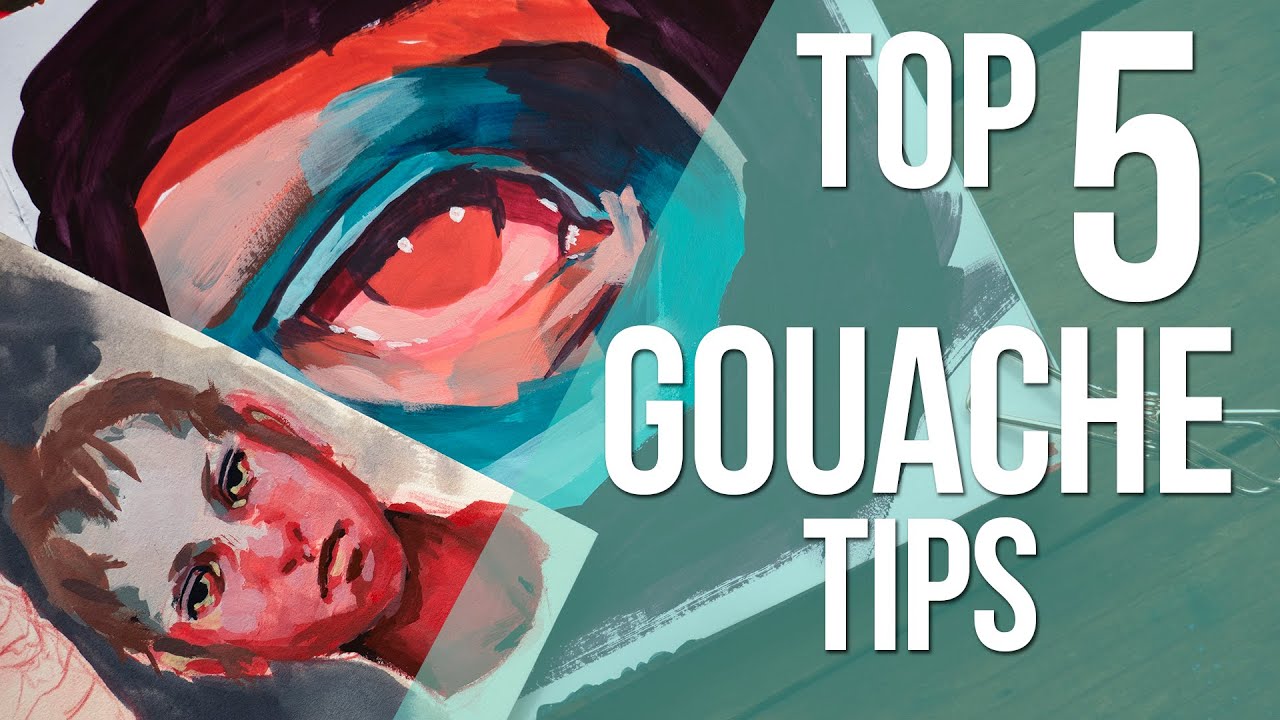The image features a rectangular illustration split into two sections. On the right side, there is bold, uppercase white text that reads "TOP 5 GOUACHE TIPS," with a muted blue, almost translucent background that fades into a gradient. This background has an underlying wooden texture subtly visible through the blue hues. The text occupies a significant portion of the right half of the image, contributing to an artistic and educational aesthetic.

On the left side, there is a striking painting of a boy's face, rendered with a mix of reddish and blue tones. The boy has brown hair, and his head appears tilted slightly, giving the image a dynamic composition. Above this, there is a close-up of an eye, characterized by a red iris, blue eyelids, and red eyebrows, all encased within a dark outline. Both the boy’s face and the eye exhibit a painterly style, emphasizing the artistic theme of the illustration. The entire image is stylized to convey tips related to gouache painting, blending vibrant colors and textures to draw the viewer's attention.